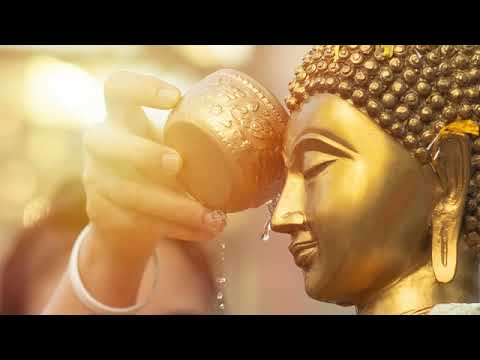The image is a small, rectangular photograph featuring a significant spiritual or religious scene. At the center-right is a golden statue, possibly representing a Buddha, characterized by its serene expression with closed eyes and a subtle smile. The statue displays intricate details: it is adorned with a beaded hat, and its ear has an elongated, drooping shape, suggesting a place for large earrings, underlined by a small hole.

On the left side of the image, a human hand with a light skin complexion, dressed in a white sleeve and wearing a white bracelet, is seen. This hand belongs to a woman, partially visible with longer brown hair but her eyes remain out of the frame. She is holding an ornate golden bowl decorated with patterns, possibly floral and leaf-like designs. This bowl is tilted, pouring water over the statue’s head.

The background is very blurred, with indistinct details, except for a hint of yellow light in the upper left corner, contributing to the overall sacred and serene atmosphere of the scene. The borders at the top and bottom of the image are solid black, creating an elongated rectangular frame for the photograph. The color image is free from any numbers or text.